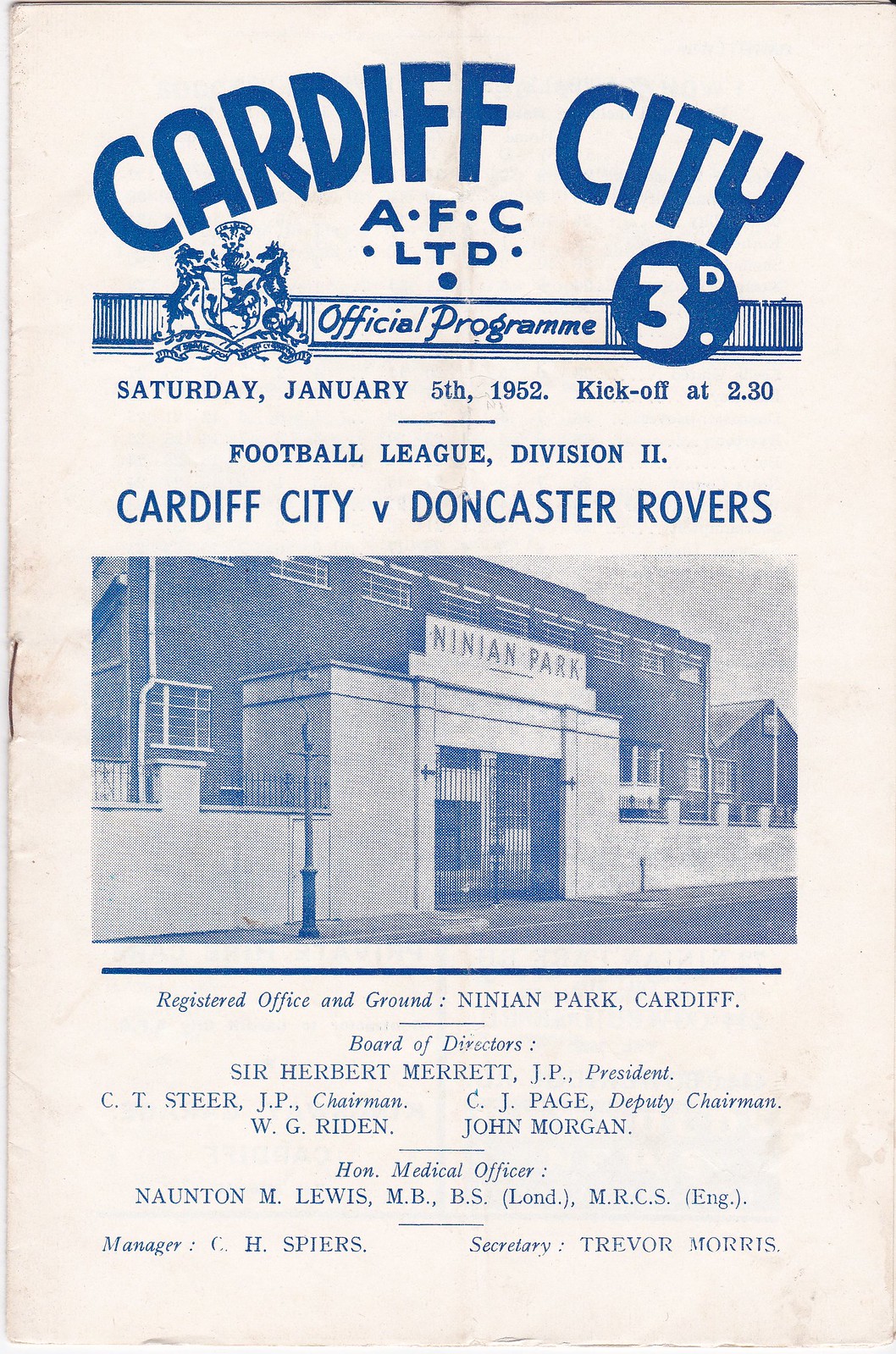This image depicts an old and worn soccer program from Cardiff City AFC Ltd dated Saturday, January 5th, 1952, with a kickoff at 2:30 PM. The cream-colored cover features prominently blue text in a semicircle at the top, stating "Cardiff City AFC Ltd." Below this, a banner announces "Official Program 3d," indicating the price. The program details a Football League Division Two match between Cardiff City and Doncaster Rovers. Central to the cover is a blue and white ink illustration of the entrance to Ninian Park stadium, with the stadium name clearly marked above the gate. The lower section of the cover provides administrative details, including "Registered Office and Ground, Ninian Park, Cardiff," followed by the Board of Directors: President Sir Robert Merritt JP, Chairman C.T. Steer JP, Deputy Chairman C.J. Page, W.G. Ridden, and John Morgan. The Honorable Medical Officer listed is Naughton M. Lewis MBBS, and the Manager and Secretary are C.H. Spears and Trevor Morris, respectively. The overall faded and worn appearance of the cover adds to its historical charm, indicating its age and the storied history of the club.